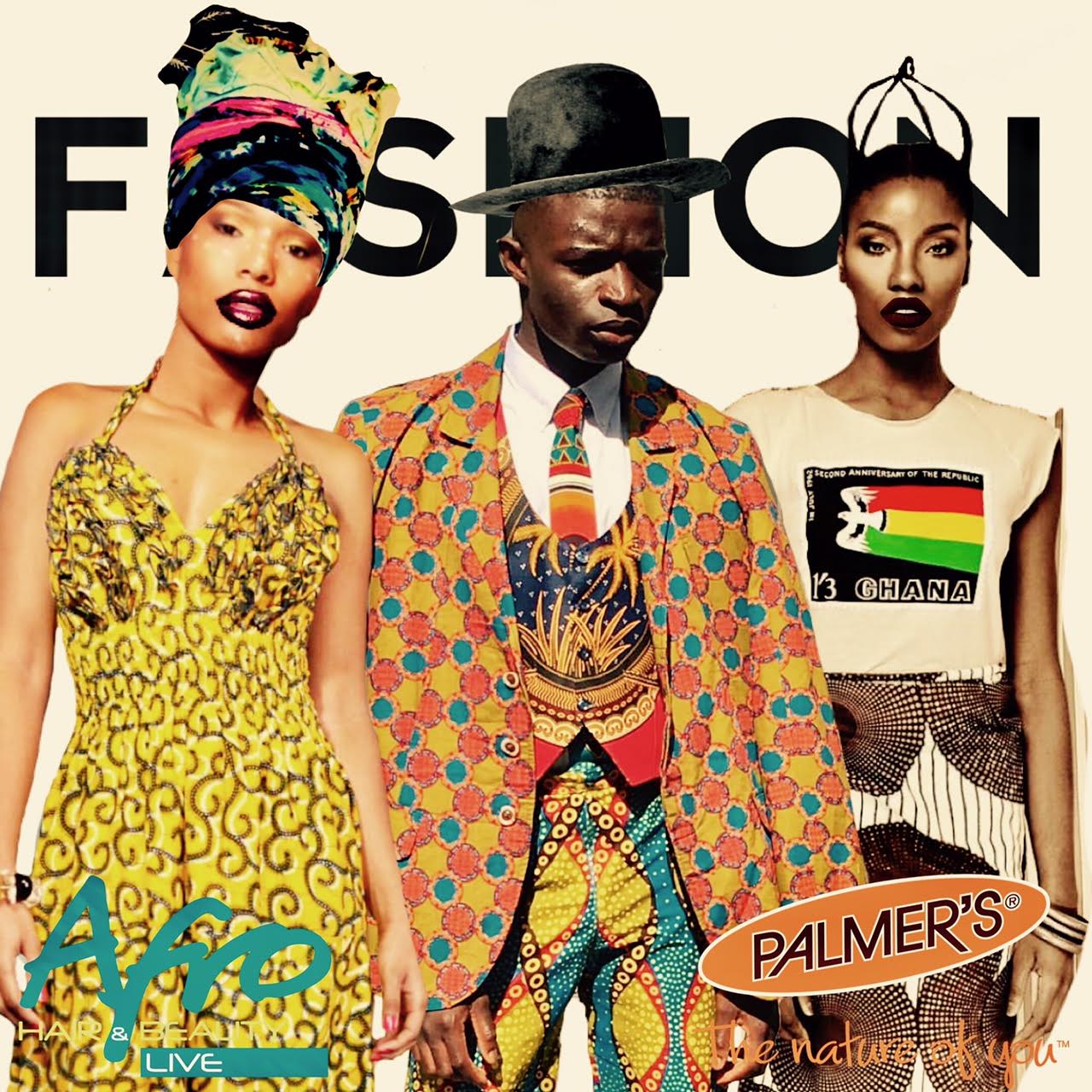This vibrant fashion photography image features three distinctively styled individuals of African descent set against a yellow-white backdrop. At the forefront, on the left, a woman is adorned in a yellow sundress with dark squiggles, completed by a colorful head wrap and dark lipstick. In the center stands a person of indeterminate gender, wearing a distinctive black bowler hat and an oversized, vividly patterned blazer in red, blue, and yellow, paired with matching brightly colored pants. The rightmost woman showcases a striking look with her hair styled into a four-braid crown, donning a white short tee emblazoned with the Ghana stamp and a bold patterned black and white dress. The bottom of the image prominently features the Palmer's logo and the tagline, "The Nature of You, TM." Additionally, the left side reads, "AFRO, Afro Hair and Beauty, Live." The top part of the image hints at the word "fashion," partially obscured by the figures.